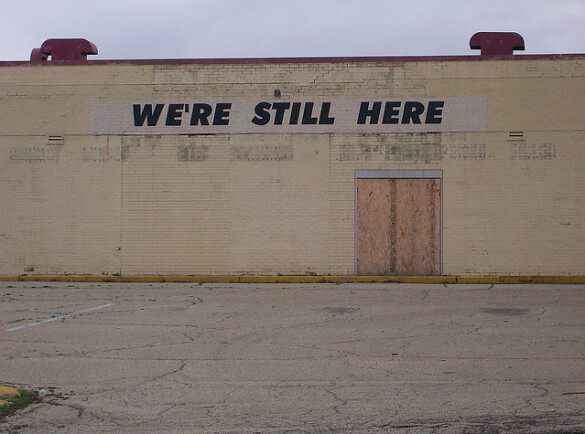The image depicts a scene with a serene, blue sky as the backdrop. Dominating the foreground is a white brick wall, featuring a wooden door with brown trim at the bottom. Above the door, a white rectangular sign with black text announces, "WE'RE STILL HERE." Interestingly, the brown trim appears predominantly gray, almost creating a sense of ambiguity between the colors. Additionally, a fine white line is visible, adding a subtle detail to the composition.